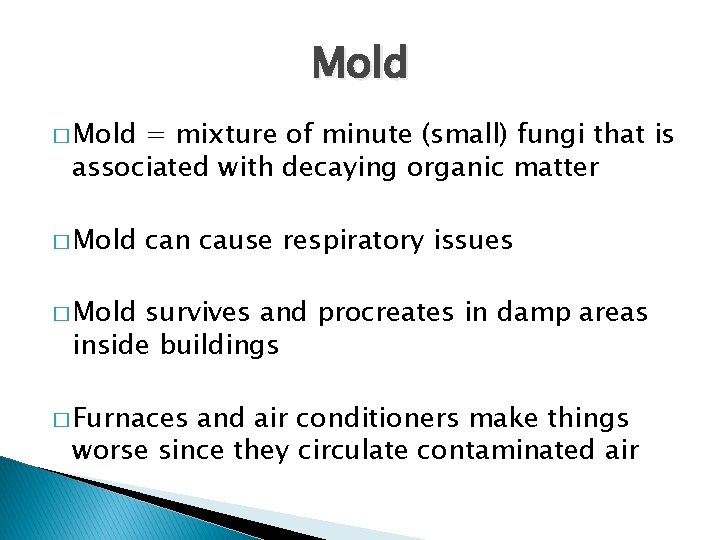The image is a detailed informational slide, resembling a PowerPoint presentation, with a white background and black text. The slide is primarily composed of text, formatted in well-positioned bullet points that are bordered by teal-colored squares. The slide's title at the top reads "Mold," and it defines mold as a mixture of minute fungi associated with decaying organic matter. Additional bullet points explain that mold can cause respiratory issues, it thrives in damp areas inside buildings, and that furnaces and air conditioners worsen the situation by circulating contaminated air. In the bottom left corner of the slide, there is a decorative blue stylized triangle element. The colors featured in the slide include white, black, light blue, turquoise, and dark gray, adding a visual structure to the content-heavy presentation.